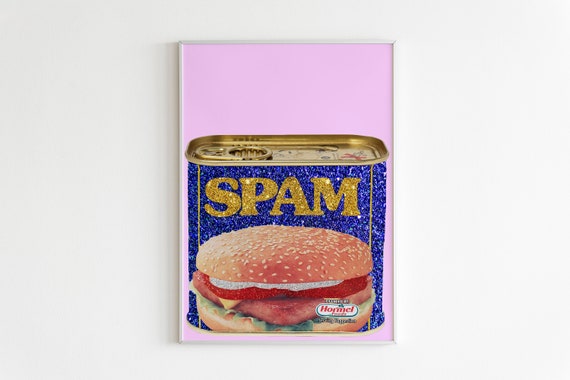The image depicts a photorealistic representation of a Spam can, situated on a pastel pink rectangular background, with a white outer frame. The Spam can is not real but rather an image of a can, rendered with a slightly glittery texture. The classic blue body of the can features the iconic word "Spam" in bold yellow letters. The top of the can has a gold aluminum pull-tab. On the front of the can, there's an illustration of a Spam sandwich comprising a sesame seed bun, Spam slices, cheese, possibly another type of red meat, tomatoes, lettuce, and other colorful elements like white, red, orange, pink, green, and yellows. The Hormel branding, located at the lower right-hand side of the can image, includes red lettering on a white backdrop. Additional text at the bottom likely provides nutritional or identification information. The rectangular pink backdrop appears to be a poster board, adding an additional layer of visual appeal to the arrangement.